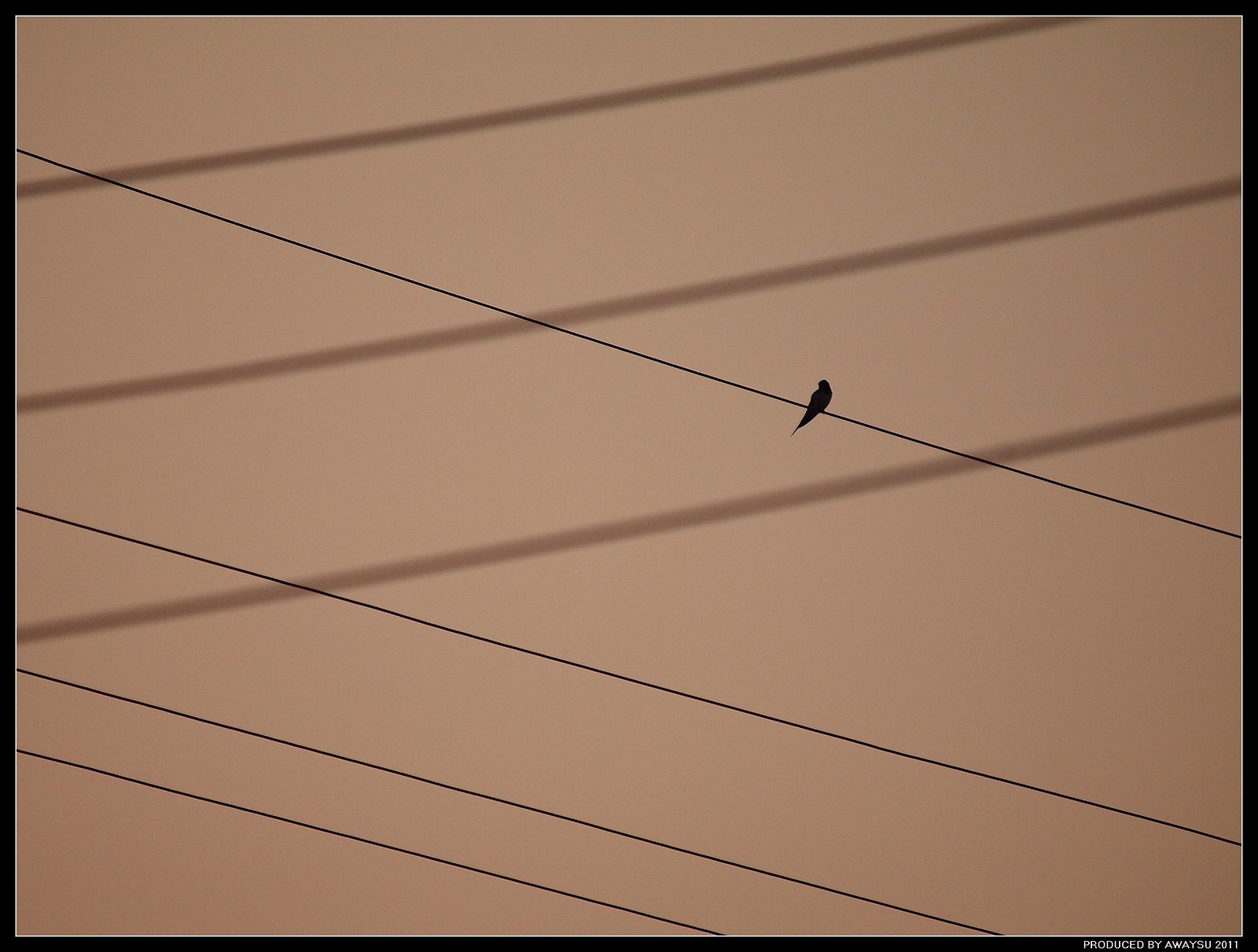The image features a black bird sitting on the top of a series of four parallel power lines that extend from the left corner to the lower right corner of the image. The bird, positioned almost centrally, gazes towards the left. The background is a tan, dark beige color, evoking a sense of a smoky or smoggy day, possibly due to wildfires. In addition to the four main wires, there are three other lines that run from the top right to the lower left, which appear to be shadows, reflections, or textures. The overall setting is outdoors, viewed from the ground looking upwards into the sky, with no additional animals, buildings, or vehicles present. The image is bordered by a black frame and in the bottom right, the text "Produced by Oasis 2011" is visible. The predominant colors are black, tan, and white.